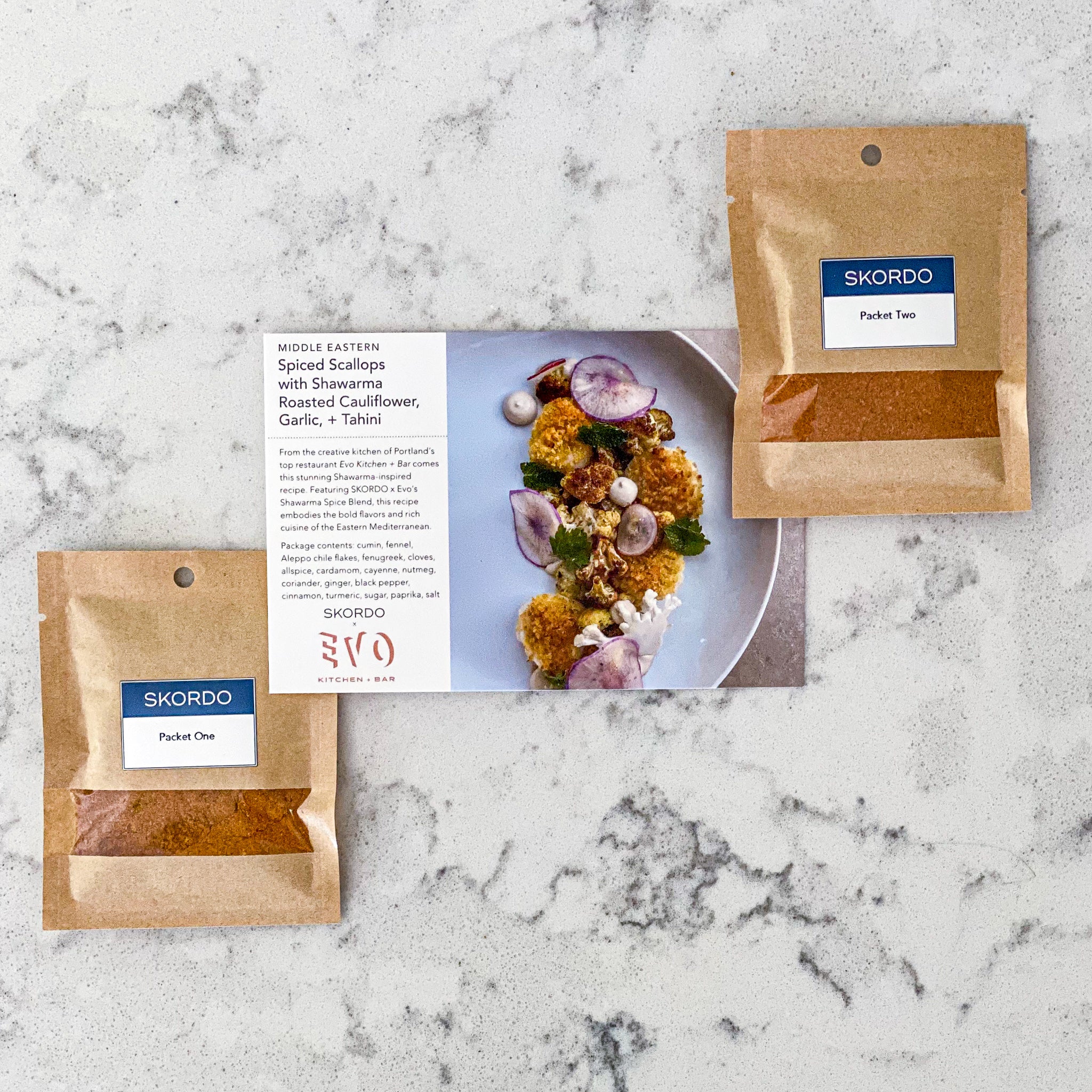The photograph features a meal kit from Skordo, displayed on a marbled gray and white countertop. Central to the image is a recipe card positioned vertically, depicting a beautifully plated dish of Middle Eastern Spiced Scallops with Shawarma, Roasted Cauliflower, Garlic, and Tahini, garnished with sliced radishes. Flanking the card are two unopened brown paper packets, each containing a cinnamon-colored spice visible through a clear plastic window. The packets, labeled "Packet 1" and "Packet 2" with blue and white labels, are strategically placed with Packet 1 positioned at the top right, slightly in front of the recipe card, and Packet 2 at the bottom left, partially covered by the card. The overall arrangement exudes an organized and inviting culinary presentation.